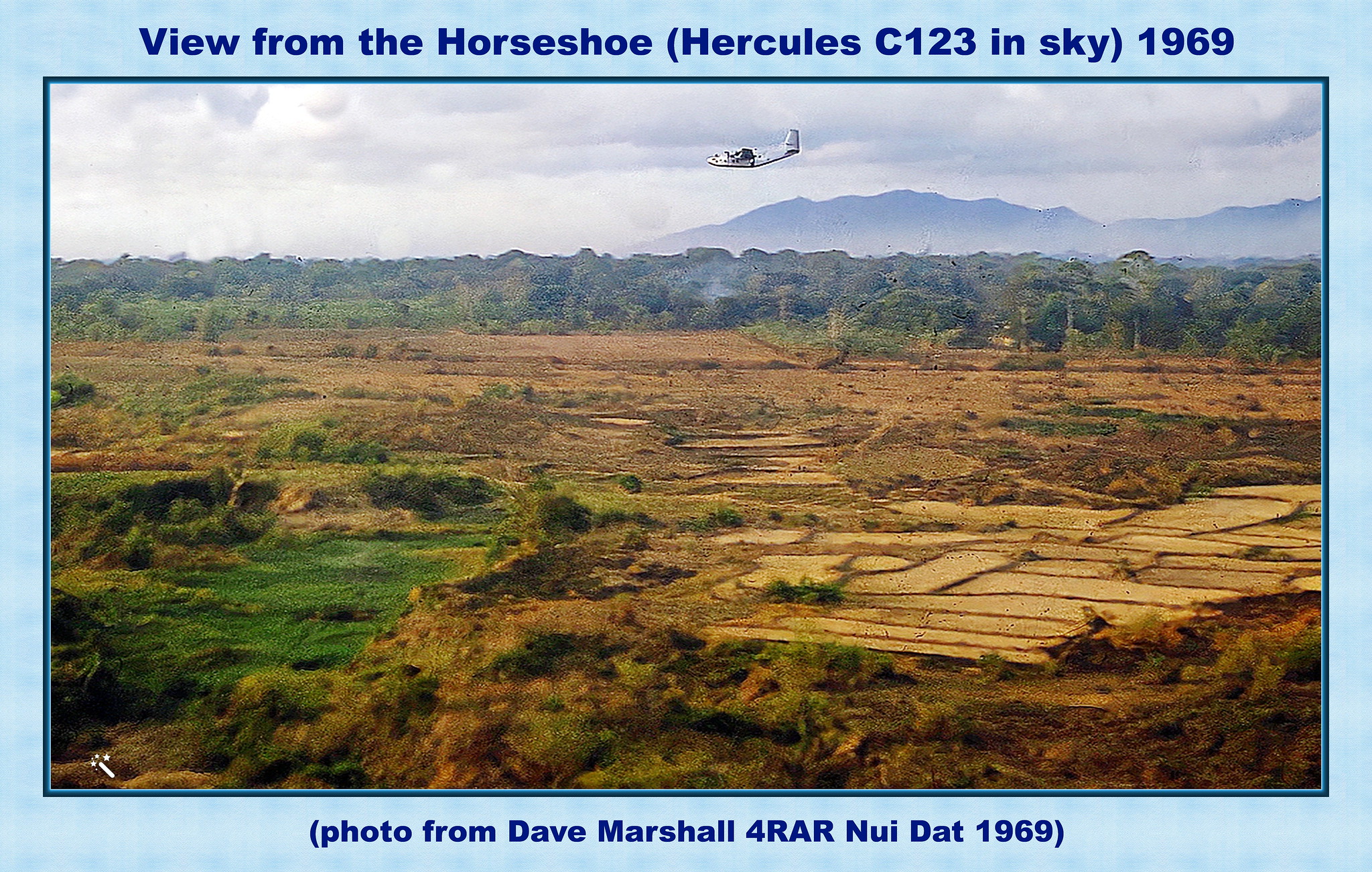This horizontally oriented, blue-bordered photograph, resembling a postcard, is labeled at the top with "View from the Horseshoe, Hercules C-123 in Sky, 1969". Below, additional text reads, "Photo from Dave Marcell, 4 RAR, Nui Dat, 1969," indicating it's a picture from Vietnam. The image prominently features a rugged field with patches of grass and divided brown dirt in the foreground. In the background, there is dense jungle transitioning to a mountain range in dark relief. A small aircraft, identified as a Hercules C-123, appears in the cloudy sky. This military photograph offers a stark view of the landscape, blending natural elements with a glimpse of wartime aviation.